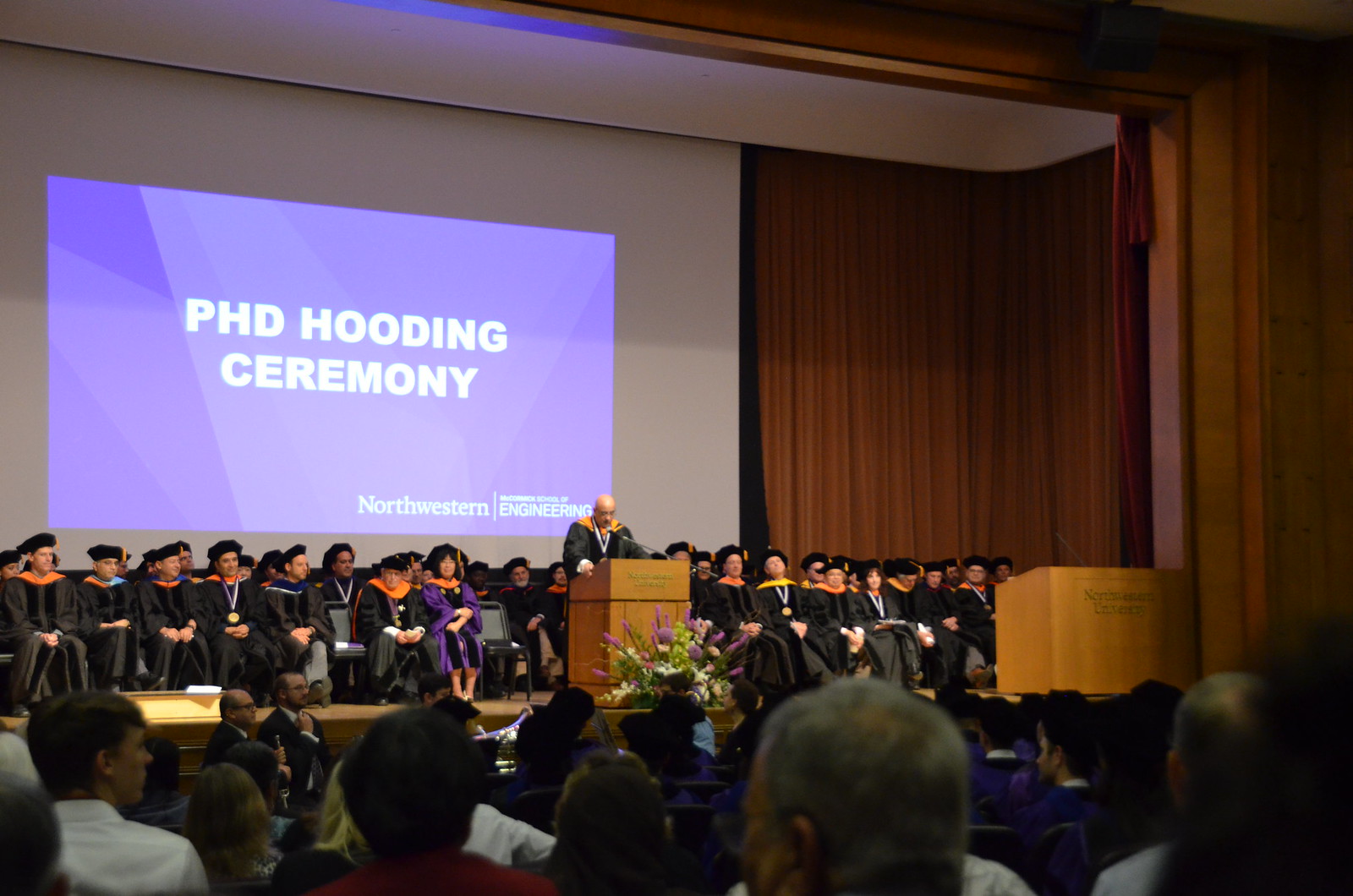The image captures a PhD Hooding Ceremony for Northwestern Engineering taking place on a dimly lit stage. At the center of the stage stands a brown podium, adorned with gold lettering that reads "Northwestern University." A man in a black graduation robe, featuring a yellow collar and a white medallion around his neck, is speaking at the podium. His bald head is uncovered, contrasting with the mortarboards worn by the other graduates. Behind him, approximately 50 individuals are seated, dressed in black graduation gowns with various colored collars, including orange, yellow, and blue. A large illuminated screen behind them glows purple and bears the text, "PhD Hooding Ceremony, Northwestern Engineering." In front of the stage, the audience members can be seen, though details are obscured due to the dim lighting, sparking a sense of solemnity and anticipation in the ceremony.